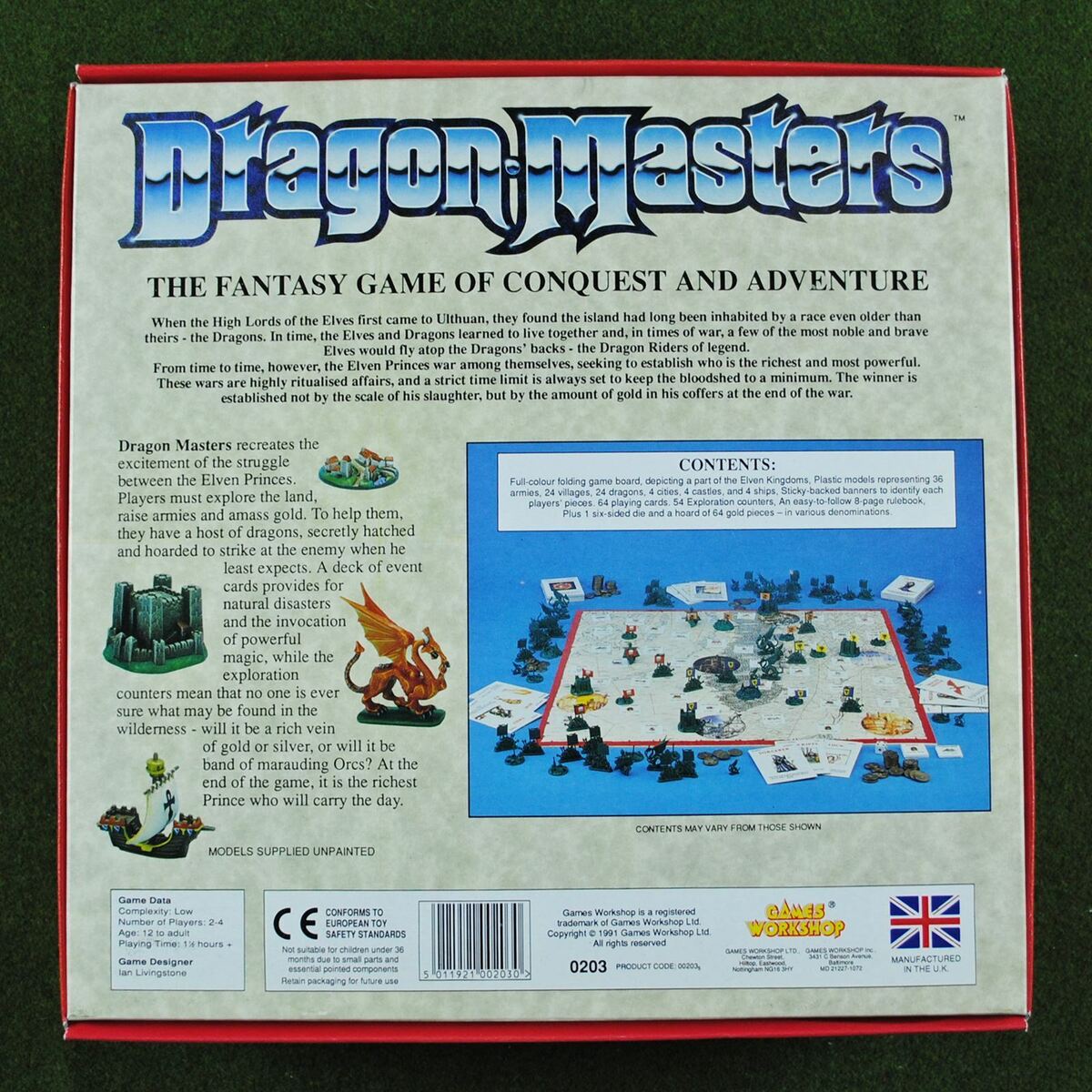The back of the game box for "Dragon Masters" is detailed and visually rich. At the top in blue letters, the title "Dragon Masters" is prominently displayed, with the subtitle "The Fantasy Game of Conquest and Adventure" in black beneath it. The text describes the game as one of strategy, where players recreate the excitement of ancient struggles between Elves and Dragons. Players must explore the land, raise armies, and amass gold, with dragons secretly hatching to strike at enemies. Highlighted text narrates the history of the Elves and Dragons on Uhtuan and the ritualized wars between Elven princes, who vie for wealth and power.

The left side of the back features images of various game pieces, including a small gray castle, a dark-colored Viking ship with a white flag, and a small dragon. The right side showcases a picture of the game board fully laid out, surrounded by cards and various pieces, indicating the game's intricate layout. The game board itself is tan with a white border, and the pieces come in various colors. At the bottom, there's a barcode, a British flag indicating manufacture in the UK, and information about the company Game Workshop, including a note that it conforms to European toy safety standards and is a trademark of Game Workshop LTD, dated 1991. The overall coloring of the box is tan, with a blue background for the photo insert.